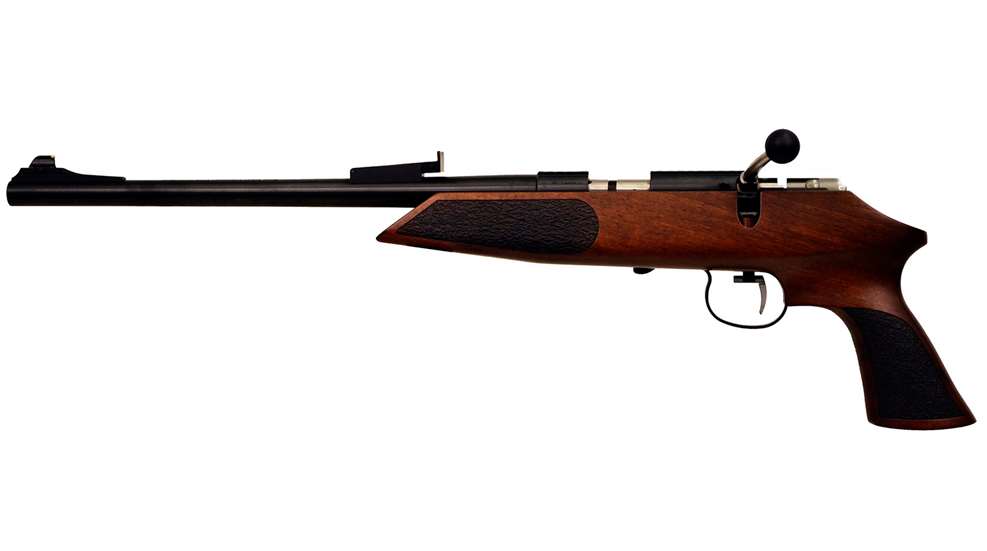In this side view image, we see a bolt-action pistol with a long black barrel, equipped with both a front sight and a rear sight for aiming. The barrel is sleek, accentuating the firearm’s precision capabilities. The handle is constructed from deep cherry-colored wood, featuring black grip panels on the sides and front for a secure hold. The trigger guard and trigger are black, fitting seamlessly into the functional design of the gun. Notably, the bolt-action mechanism is visible but not pulled back. The firearm, designed for one or two-handed use, is pointing to the left side of the image, showcasing its detailed craftsmanship and mechanical components.